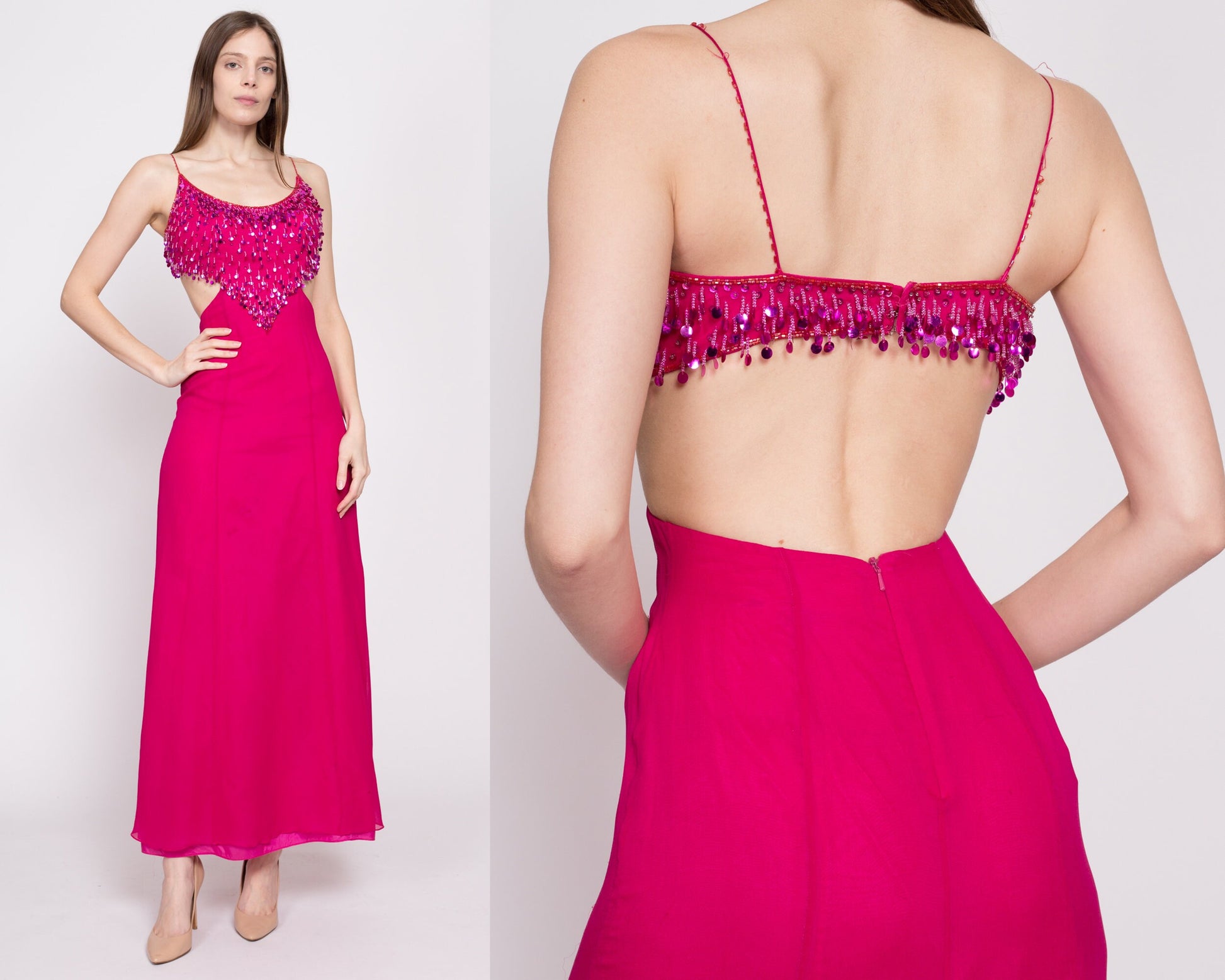The image features two vertically aligned photographs of the same woman, presented side-by-side against a plain white background. The left image, occupying about one-third of the total width, is a full-body shot showcasing the woman standing tall and confident. She has long brown hair cascading down her back, pale skin, and is wearing a striking long pink dress adorned with thin shoulder straps. The dress features intricate beading around the chest and upper body, which catches the eye with its sparkling detail. Her right arm is poised on her hip while her left arm rests naturally by her side. She completes her look with tan-colored high heels.

The right image, taking up approximately two-thirds of the total width, offers a close-up rear view of the same woman. This photograph highlights the delicate design of the back of her dress, which exposes her upper back and is fastened with a zipper. The beaded detail continues at the back, with a pink band running horizontally across the center of her back, giving a glimpse of her skin below. Her arms are positioned in front of her body, adding to the elegant and sophisticated appearance portrayed in both images.